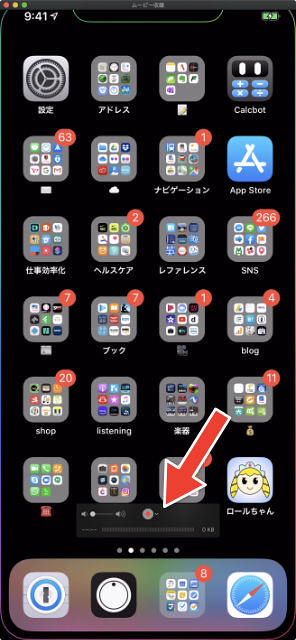This image depicts a screenshot of an iPhone's home screen. The screenshot is slightly blurry and of low resolution. The background color of the screen is black. In the top left corner, there are three circular icons: a red circle, followed by a yellow circle, and then a green circle. Centered at the top, there are Japanese characters displayed in white. Directly below the colored circles, there is a number sequence "941" in white text. In the top right corner, a green and white battery icon indicates the phone's battery status.

The home screen shows numerous app icons, though details are not clear due to the image quality. In the upper left area of the screen, there is an app with a square, gray icon that features a black and gray gear symbol, indicating the Settings app.